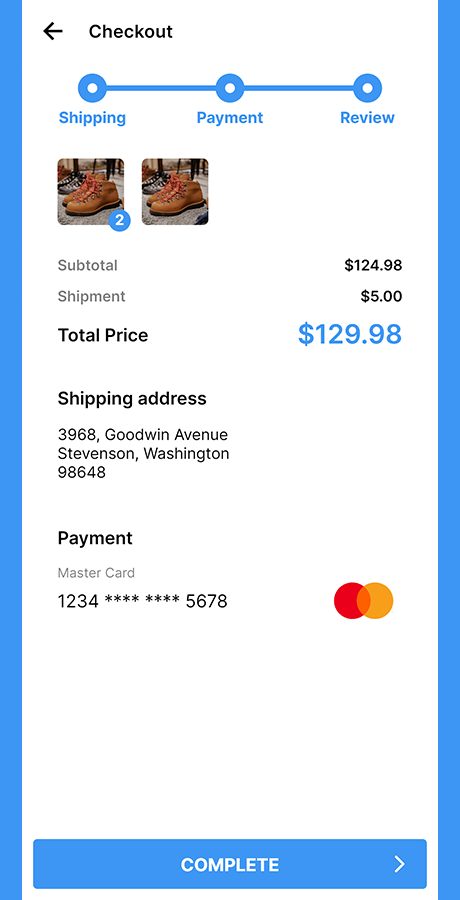The image captures a screenshot of a checkout page viewed on a cellphone. At the top left corner, the word "Checkout" appears in black font next to a left-pointing arrow, also in black. Just below this, there is a small progress line indicating that a product has been shipped, and the payment is being reviewed.

Moving downward, the display shows two identical pictures of brown work boots, featuring both low-top and high-top styles with distinct red shoelaces. The total price for the boots is $129.98, with a shipping cost of $5.00, bringing the subtotal to $124.98.

The shipping address listed is 3968 Goodwin Avenue, Stephenson, Washington, ZIP code 98648. The payment method used is a MasterCard, with half of the card number obscured by asterisks for security. To the right of the payment details, the MasterCard logo, consisting of two overlapping circles—one light yellow and the other red—is clearly visible.

At the bottom of the screen, a large blue rectangular button is displayed, labeled "Complete" in white text. The entire page has a blue border background, framing the checkout information neatly.